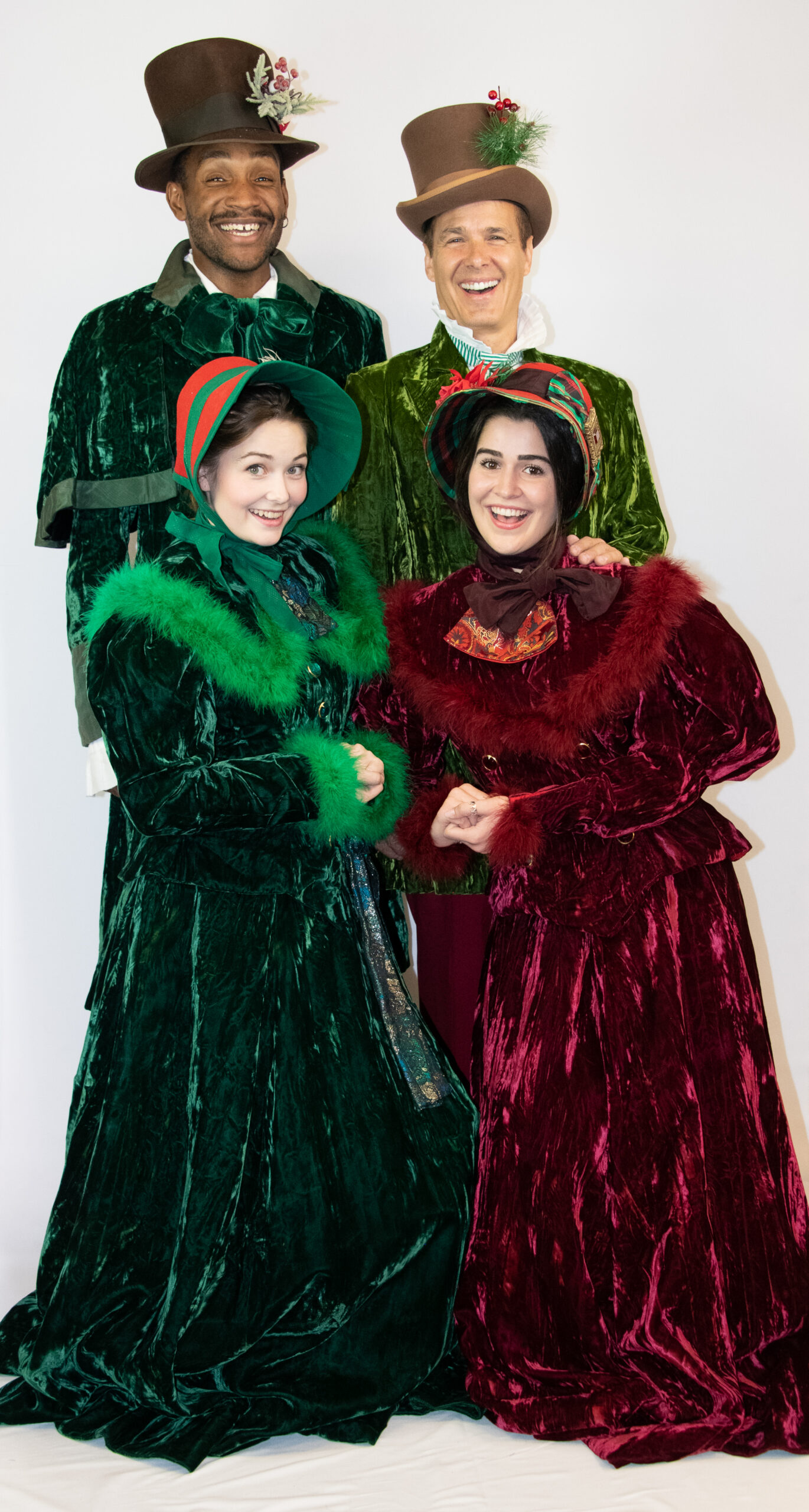The image depicts four individuals posing together for a photo, likely intended as a humorous Christmas card. The group consists of two men and two women, with the women positioned in front of the men. The setting is a white background, emphasizing the distinct, festive attire of each person, which evokes a late 1800s theme.

Starting from the left, the man is dressed in a dark green velvet suit paired with a black top hat adorned with a sprig of mistletoe bearing red berries. He wears a green bow tie and underneath the suit, a white collared shirt is visible. This man is smiling brightly, adding to the cheerful atmosphere. The woman next to him wears a long, heavy dark green velvet dress with fur trim around the collar and wrists. She also has a plaid green bonnet decorated with red and dark brown stripes.

To her right, the man behind her is clad in a lighter green outfit, somewhat lime green, and a brown top hat also featuring a mistletoe sprig with berries. His attire includes a velvety top and a white collared shirt, contributing to the holiday spirit. He, too, wears a broad smile that enhances the joyful mood of the picture. 

Lastly, the woman on the far right stands out in a deep dahlia purple velvet dress, which has a slight pinkish hue, and similar fur trimmings at the collar and wrists. She wears a bonnet adorned with red and green colors, though the exact details are obscured. Both women have bonnets tied under their chins, likely accented with bows, and they share a warm smile, complementing the men’s lively expressions in the background.

Together, their matching smiles and elaborate period costumes, complete with top hats and bonnets, make for a whimsical and festive group portrait.